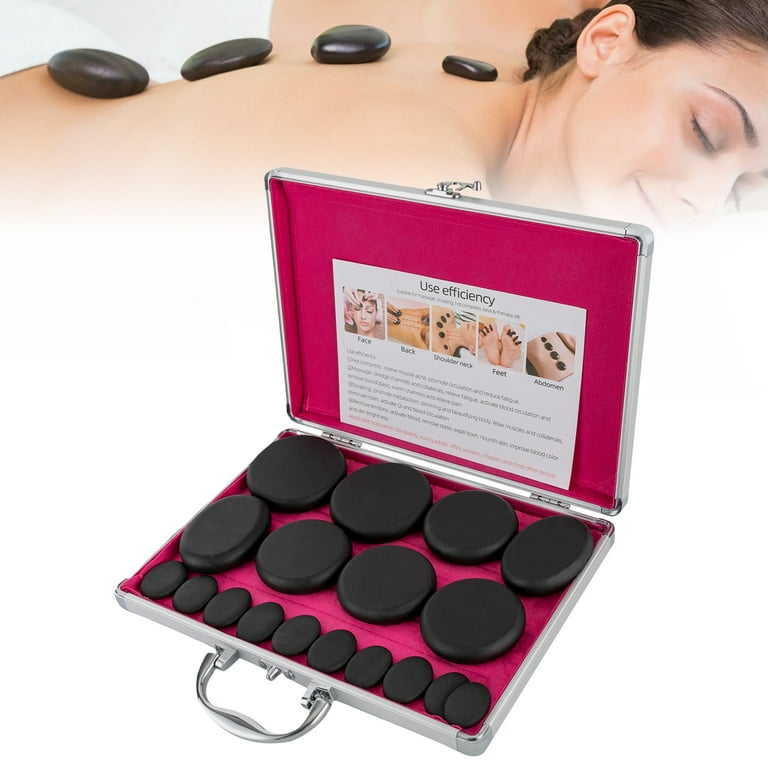The image vividly depicts a comprehensive hot stone massage kit, featuring an open chrome briefcase with a pink felt interior. The lower section of the case neatly organizes eight large circular black stones in one row and a series of smaller oval stones in another. The inside lid of the case contains detailed usage instructions alongside illustrative images demonstrating the stones' application on various body parts, including the face, back, shoulders, neck, feet, and abdomen. Above the briefcase, a serene, semi-transparent image of a woman lying face down with her eyes closed is shown, smiling softly as a series of polished black stones are strategically placed along her spine, increasing in size from the lower to the upper back. The overall setting of the image is clear and bright, benefiting from natural lighting that enhances the clarity and color of the scene, making it evident that this kit is intended for spa treatments and massages, possibly for sale online.